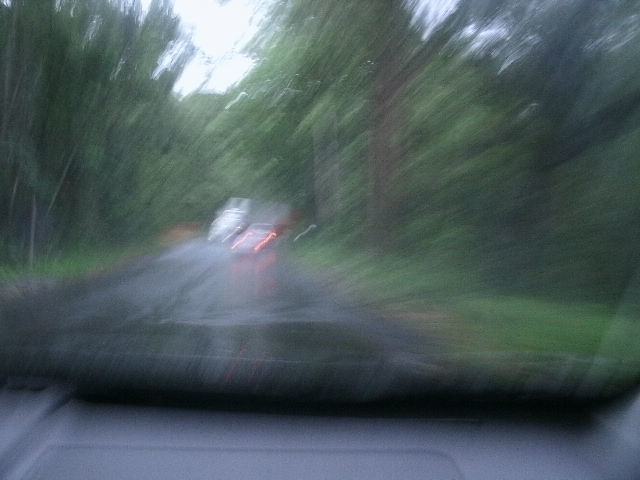The image is a very blurry photograph taken from the passenger side inside a moving car. The picture captures a scene on a narrow, forested, one-lane road or highway. You can make out the car's dashboard at the bottom, with a bit of the black hood visible as well. Ahead in the distance, the taillights of a few cars are visible, appearing streaked and stretched due to the blur, giving the impression that they are shifting towards the right. On the opposite side of the road, there is a white semi-trailer truck approaching. The surroundings are lush with thick green trees on both sides of the road, with a hint of blue sky peeking through at the top. The overall image is significantly blurry, rendering a sort of dreamy, almost rainy effect, though it may just be the result of the motion blur.